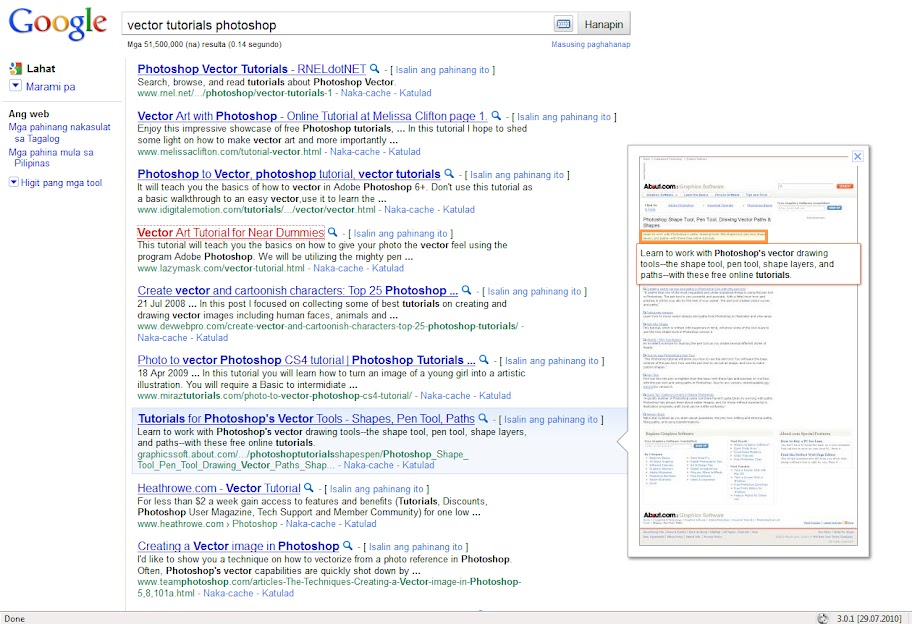The image displays a Google search results page. The familiar multicolored "Google" logo is prominently positioned at the center top. Inside the search bar, there is the query "Vector Tutorial Photoshop." Below the search bar, the results are listed.

The first three search result titles are in blue, underlined, presumably links, with descriptions in black text and additional information in green and blue. The fourth search result stands out with its red title, followed by text in black, green, and blue. Subsequent results return to the standard blue titles with corresponding black, green, and blue descriptions.

Underneath the Google logo, there's a colorful symbol, indistinct but accompanied by the text "LaHat." There is also a square icon with a downwards-pointing arrow, adjacent to some words that are too small to discern, along with black text that is similarly indiscernible. 

On the right-hand corner of the page, there's a gray-outlined rectangle with a triangular notch on the left side. Within this rectangle, small text is visible in black, orange, and blue, though it's too tiny to read.